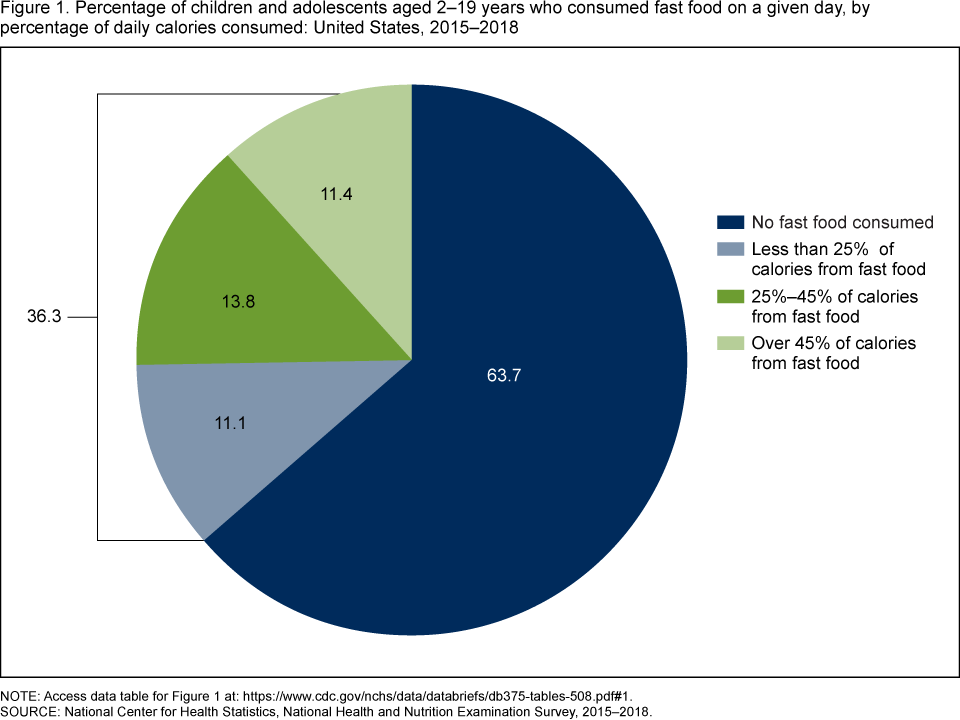The image is a detailed pie chart titled "Figure 1: Percentage of Children and Adolescents Aged 2 to 19 Years Who Consumed Fast Food on a Given Day by Percentage of Daily Calories Consumed in the United States from 2015 to 2018." The pie chart, which is featured in the center of a textbook page, is divided into four segments, each represented by different colors. The largest segment, in dark blue, shows that 63.7% of children and adolescents did not consume any fast food. The remaining 36.3% is divided into three categories: less than 25% of daily calories from fast food (light blue-gray, 11.1%), 25% to 45% of daily calories from fast food (mossy green, 11.4%), and over 45% of daily calories from fast food (light green, 13.8%). A legend on the right side clarifies these colors and percentages. Additionally, a note at the bottom of the figure provides a link to the data table and identifies the source as the National Center for Health Statistics' National Health and Nutrition Examination Survey from 2015 to 2018.